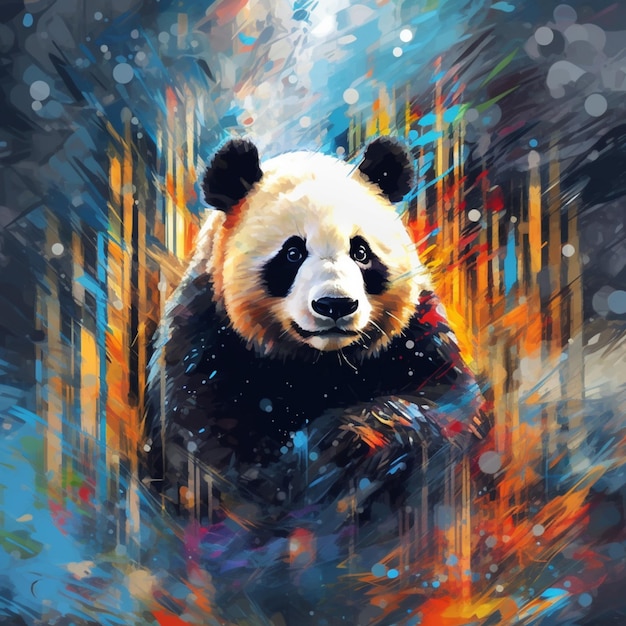The digital painting features a centrally placed panda, sitting on its back haunches. The panda exhibits classic bear-like attributes with a white face, black eye spots, and round black ears. The panda's body transitions into black fur below the neck, though the visualization of its front claw is somewhat cut off and distorted. The background is an artistic blend of hard orange lines with interspersed blue strokes, and various circles in gray and blue, contributing to a dynamic and somewhat chaotic aesthetic. Additionally, there's a small green circle with blue water and green continents, likely representing the Earth, situated in the bottom-left corner. The background also incorporates top corners painted in dark gray shades, creating a stark contrast. Elements that resemble bamboo rods and white dots, hinting at snowfall, add depth to the visual narrative. Overall, the image conveys a striking mix of colors and textures, blending sharp lines and soft splatters to create an intricate digital artwork.